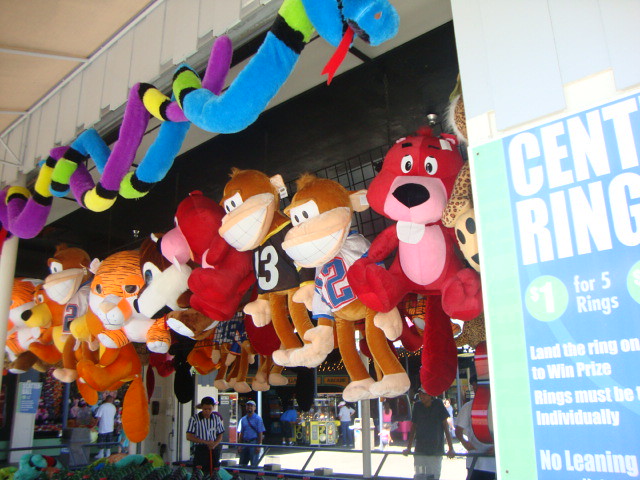The image captures a lively scene from a carnival booth adorned with an array of colorful plush animals. Along the top, vibrant snake plushies in purple with yellow and black, and blue with lime green and black, dangle enticingly. Below them, a metal grid is festooned with smiling stuffed animals, including tigers and monkeys wearing sports jerseys. Additional characters like a fox with a large tail and a beaver with buck teeth add to the variety. The background reveals a bustling marketplace atmosphere with people milling around, sunlight illuminating the scene. A man dressed in a referee shirt is visible, enhancing the festive ambiance. On the right side, a partially visible blue sign with white text offers carnival game instructions: "One dollar for five rings. Land the rings on to win a prize. Rings must be individually. No leaning."